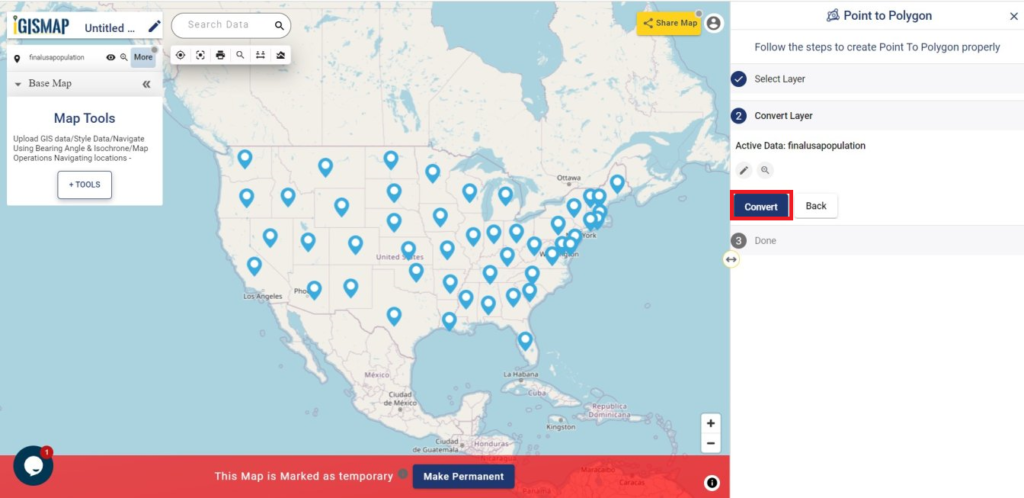**Title: Interactive GIS MAPHS Webpage Displaying U.S State Capitals**

**Description:** The image depicts a detailed webpage showcasing an interactive Geographic Information System (GIS) map known as MAPHS. This map meticulously highlights the capitals of each U.S. state, represented by numerous blue location dots strategically placed across the country. The user's interface is designed for easy navigation and searchability, featuring a prominent title "GIS MAPHS" adjacent to a rounded search box. A clickable magnifying glass icon within the search box allows users to efficiently search for specific locations.

**Features:** Below the search box, there is an additional function panel containing options like "Base Map" and "Map Tools", with "Map Tools" highlighted in blue. 

**Map Details:** The map itself illustrates the United States in a light whitish hue, clearly delineating state borders, and extends to show surrounding countries, including Canada and Mexico, as well as neighboring lakes and oceans in a light blue shade. 

**Note:** At the bottom of the webpage, a red bar states, "This map is marked as temporary, make permanent," indicating a prompt for the user to confirm the map's status. This comprehensive visual representation facilitates an intuitive understanding of U.S. geography and state capitals.